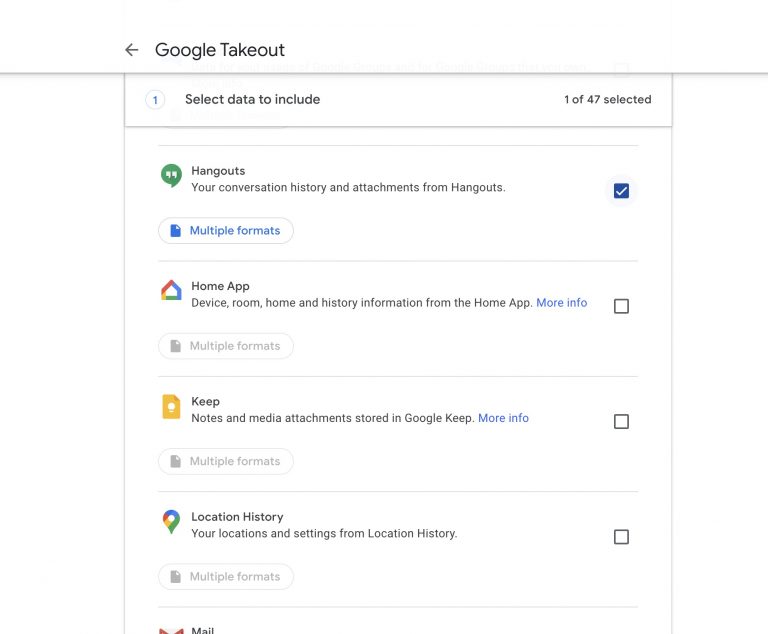The image shows a Google Takeout interface. 

In the upper left corner, the text "Google Takeout" is displayed in black, with a left-pointing arrow beside it. A gray line runs below this section. Beneath the line, the header "Select data to include" appears, with "1 of 47 selected" indicated below it.

The first option on the list is "Hangouts," followed by the description "Your conversations, history, and attachments from Hangouts." This option is selected, as indicated by a blue box with a white checkmark on the right side. Below this, the text "Multiple formats" is written in blue on a white background, enclosed by a gray line.

A subsequent gray line separates this from the next option, "Home app device, room, home, and history information from the Home app." The phrase "More information" appears in blue. This option is not selected, and the accompanying "Multiple formats" text is gray.

Further down, another gray line leads to the "Keep" section, which describes "Notes and media attachments stored in Google Keep." The text "More info" is blue, but the selection box here is empty, and "Multiple formats" is gray.

The "Location History" section follows, detailing "Your locations and settings from Location History." This option is also not selected and contains gray "Multiple formats" text.

Visible below is the edge of the next option, presumably "Gmail." 

The dominant colors featured in the interface are gray, black, white, blue, green, yellow, and red.